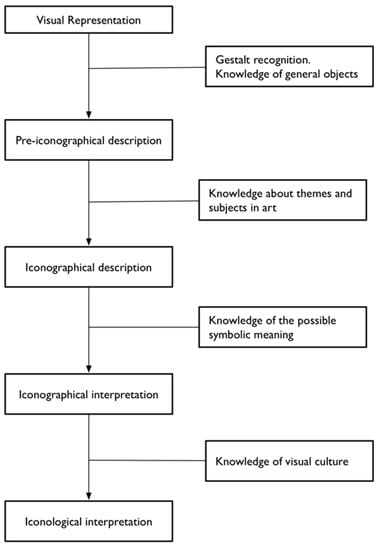The image is of a detailed flowchart consisting of multiple horizontally oriented rectangles, all outlined and lettered in blue, connected by straight-arrow lines. At the top, the first rectangle is labeled "Visual Representation," with an arrow pointing to a subsequent rectangle below that reads "Pre-iconographical Description." Continuing downward, the next rectangle is labeled "Iconographical Description," followed by "Iconographical Interpretation," and then "Iconological Interpretation." Midway between the top two rectangles, another rectangle labeled "Gestalt Recognition, Knowledge of General Objects" is connected by a horizontal line veering to the right. Similarly, between each subsequent pair of rectangles on the left, there are additional rightward horizontal lines leading to rectangles that denote "Knowledge of Themes and Subjects in Art," "Knowledge of Possible Symbolic Meaning," and "Knowledge of Visual Culture." This structured layout illustrates the progressive levels of visual and iconographical interpretation and the related knowledge necessary at each stage.